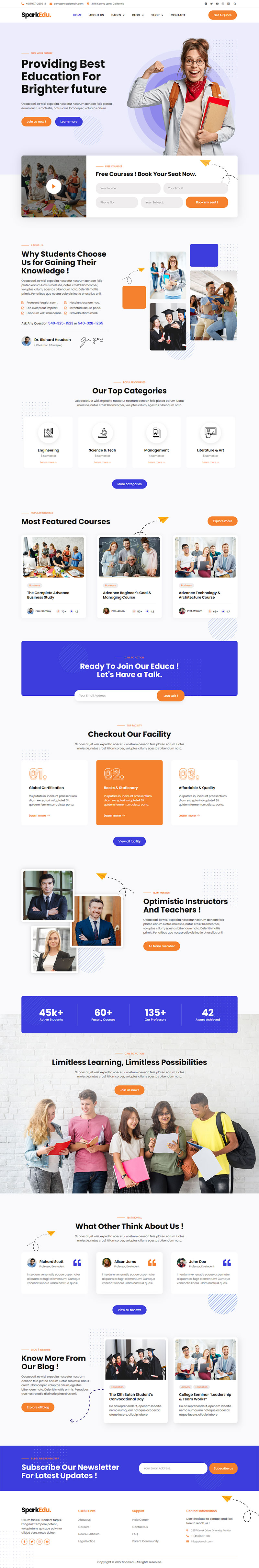The image is blurry no matter the zoom level. In the top right corner, there is a person wearing an orange shirt. To the left of this person is a text box, and below it are an orange button and a blue button. Beneath these buttons is a picture with accompanying text to its right. To the right of this section are two orange boxes and one blue box, with another blue box directly below them flanked by two orange ones. Below this arrangement is a large blue rectangular box, followed by a smaller orange box. Further down, there are three thumbnail images on the left. At the bottom of the image, there is a large picture stretching from left to right, depicting five people looking at the camera, with an orange box above the person in the middle. Below this large image are two additional pictures, with a blue box at the very bottom.